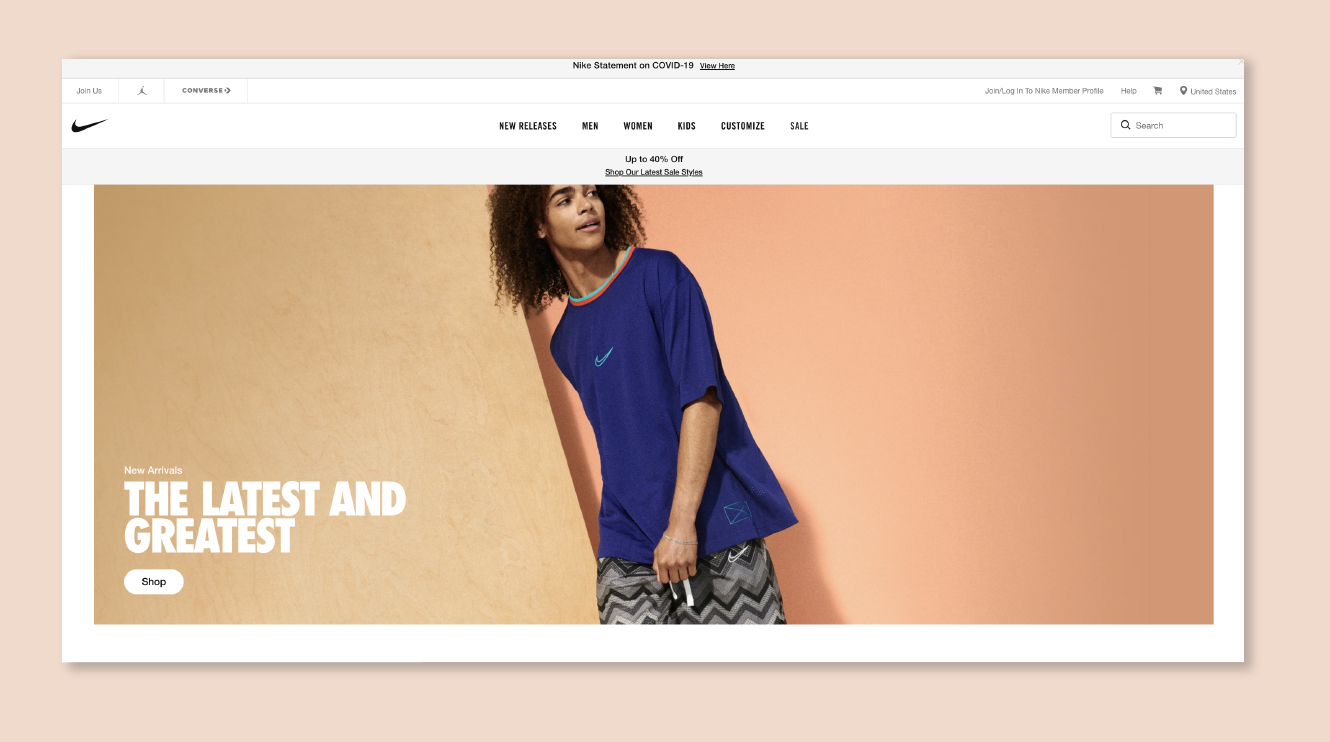The webpage features a striking image of a young male model donning a crew neck, short-sleeved Nike t-shirt in a deep, almost royal blue hue. The t-shirt is accentuated by a vibrant red and gray stripe at the neckline and prominently displays the iconic Nike swoosh in light blue on the chest. The individual has dark skin and sports long, kinky hair, adding to the dynamic visual appeal. They are captured looking over their left shoulder while holding an indistinct object in their left hand.

Completing the ensemble, the model wears edgy gray and black zigzag-patterned bottoms, although it's unclear whether they are pants or shorts due to the image cropping. The overall look is casual yet fashionable, perfectly embodying Nike's athletic and modern aesthetic.

The left side of the page features an advertisement proclaiming "New arrivals, the latest and greatest," accompanied by a clickable "Shop" button. The top of the photo is bordered by a navigation strip listing categories: "New Releases," "Men," "Women," "Kids," "Customize," and "Sale." Directly below, a banner announces "Up to 40% off, shop our latest sale styles," enhancing the shopping experience with tempting deals. This vibrant landing page is part of Nike's online store, showcasing their latest apparel and enticing customers with new and discounted items.